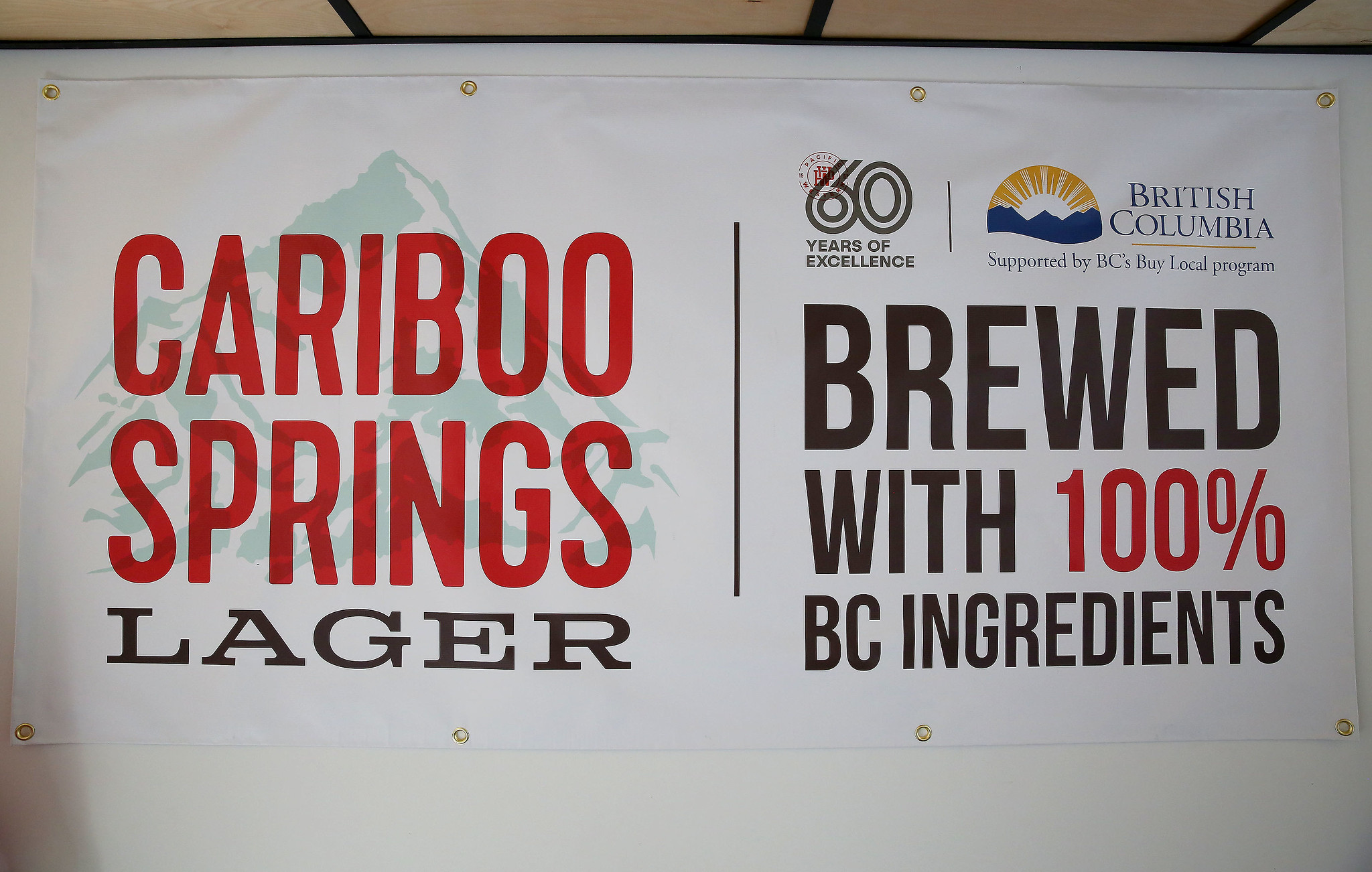This photograph captures a large promotional banner advertising Caribou Springs Lager. The banner is attached to a white wall using eyelets, and the top of the image includes a suspended ceiling. Dominating the left side of the banner are the words "Caribou Springs" in red, and "Lager" in black, with a faint image of a mountain landscape featuring snowy peaks in the background. Centered on the right side, the text "60 years of excellence" is prominently displayed alongside the statement "British Columbia, supported by BC's Buy Loco program." Below this, the phrase "Brewed with 100% BC ingredients" stands out, where "100%" is highlighted in red. Accompanying the British Columbia statement is a logo with a blue mountain and sun rays. The overall design underscores the beer's heritage and its commitment to using locally sourced ingredients from British Columbia.